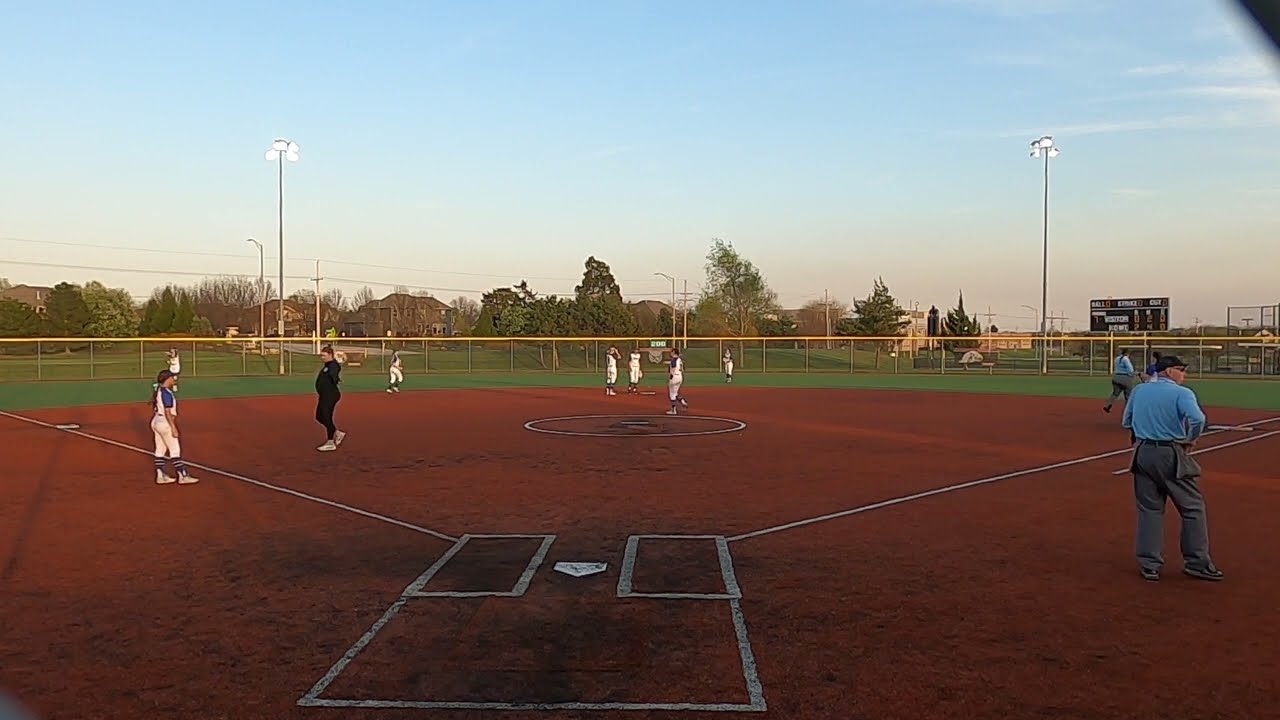The image features an outdoor girls’ softball game viewed from behind home plate. The infield showcases light red-orange dirt, meticulously lined with white markings around the bases and pitcher's mound, with white home plate clearly visible. Gathered around the diamond are players donned in white uniforms comprising white shirts and pants. In the scene’s left and center, several players stand idly, possibly conversing, indicating the game has yet to commence. On the right, an umpire in a blue long-sleeve shirt and gray pants is noticeable. Also to the right, a coach dressed in black can be seen crossing the field. Beyond the infield, stretches of lush green turf mark the outfield, bordered by a chain-link fence topped with a yellow plastic lining. In the background, the scene is framed by tall light standards, power lines, streetlights, and trees beneath a blue sky with scattered wispy clouds, evoking a pleasant evening ambiance.